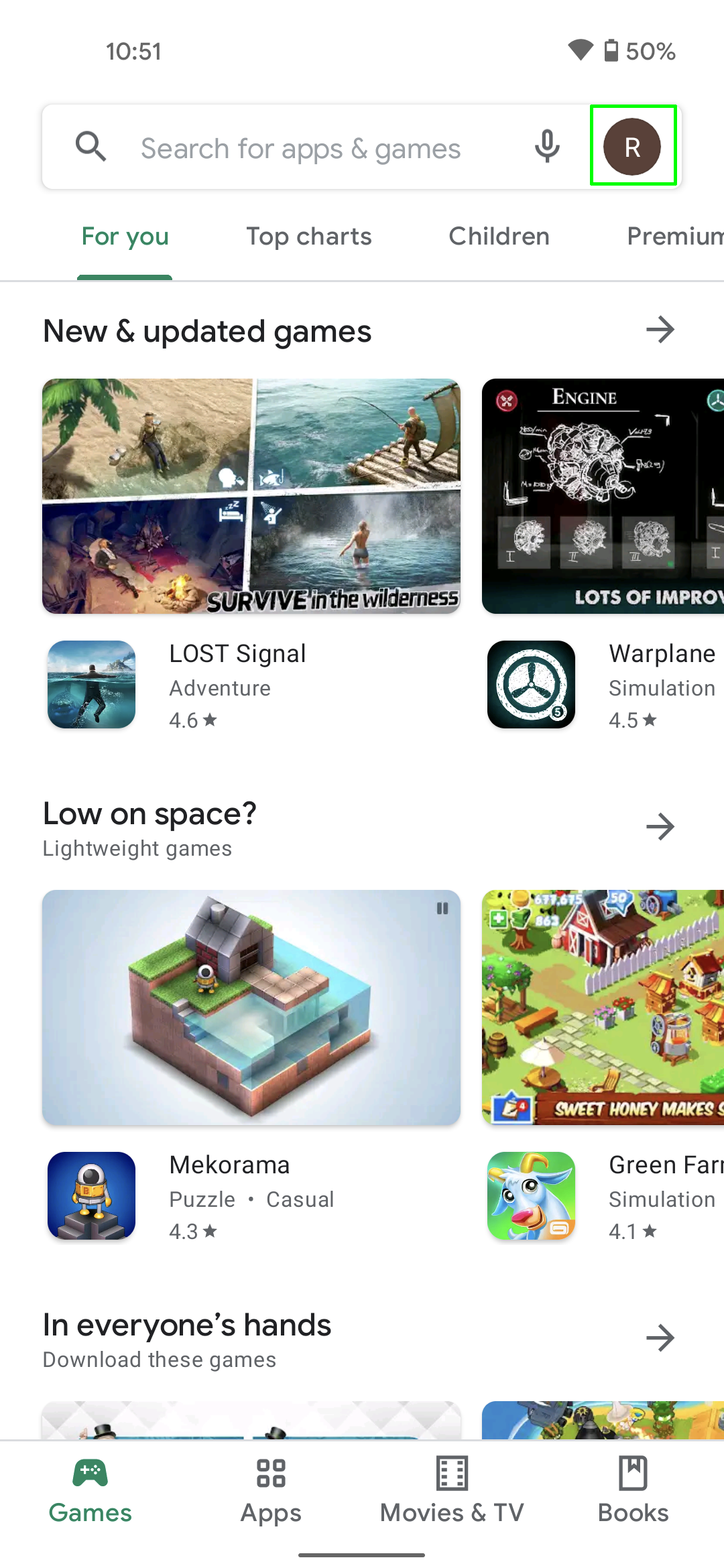This image captures a screenshot from a smartphone, predominantly featuring a white background. At the top of the screen, the time is displayed as 10:51, and the battery status, shown on the right, indicates a 50% charge. Below the time, there's a search bar labeled "Search for apps and games," accompanied by a microphone icon at its end.

To the right of the search bar, a distinct icon is visible - a white capital letter 'R' within a black circle, which is itself framed by a white square bordered in bright green.

The upper section of the screen includes a navigation tab with the options "For you," which is highlighted with darker text and an underline, "Top charts," "Children," and "Premium." Above this navigation, there is a section titled "New and Updated Games."

In this section, several game icons are displayed. The first game listed is "Lost Signal." Another game, partially visible, appears to have the name "We Planet," but is cut off, making it difficult to discern fully. Below these, more game icons are present, suggesting the possibility of scrolling down to view additional content.